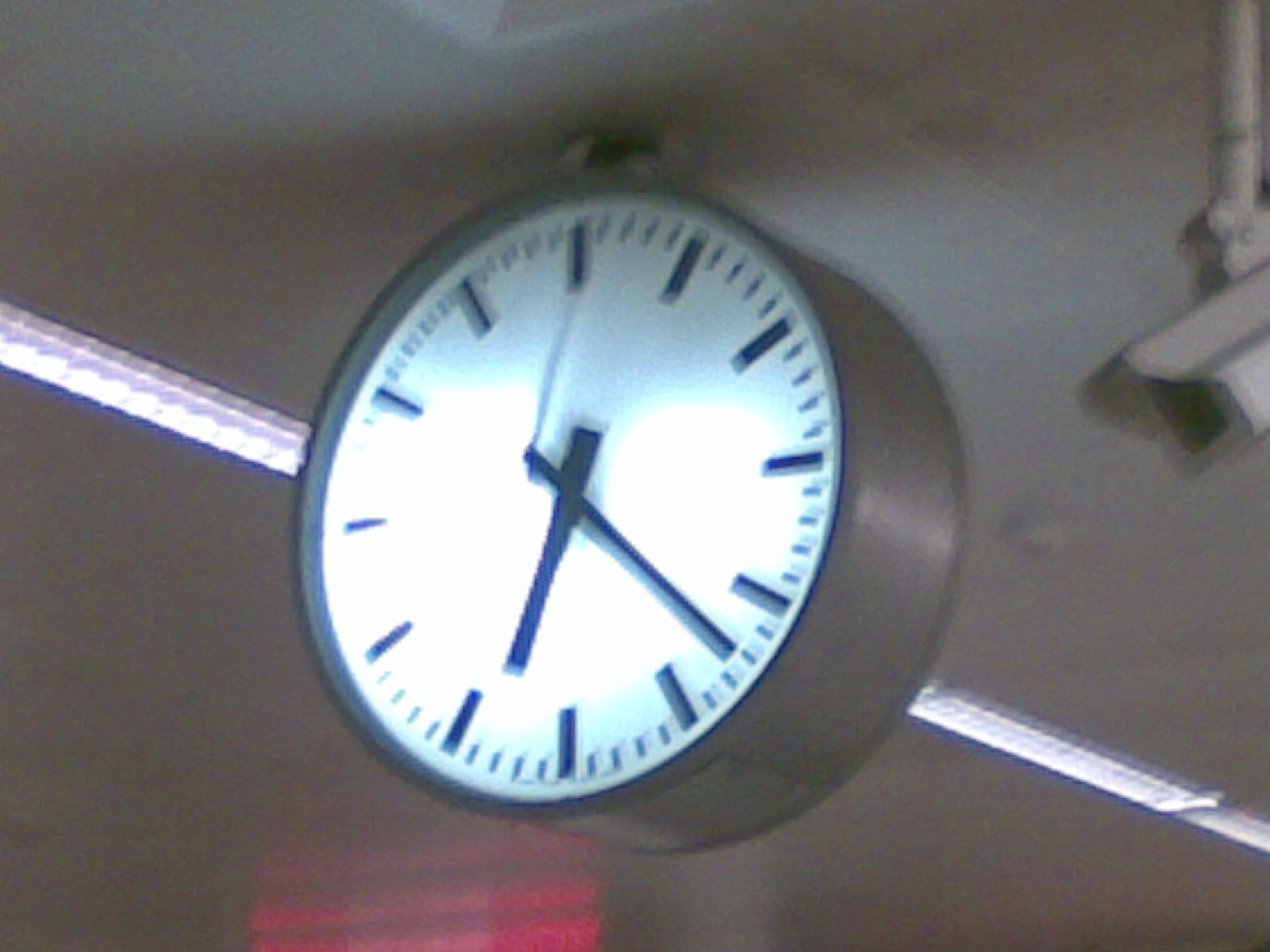This is a detailed color photograph captured inside a building. The perspective offers an elevated view, focusing on a large, round clock suspended from the ceiling. Diagonally positioned behind the clock, fluorescent lights stretch from the upper left to the lower right, illuminating the scene. The clock, with a gray casing, displays minimalistic design elements: simple black lines marking each hour and two sleek black hands indicating the time against a gray background. The overall composition emphasizes the modern, industrial aesthetic of the space.